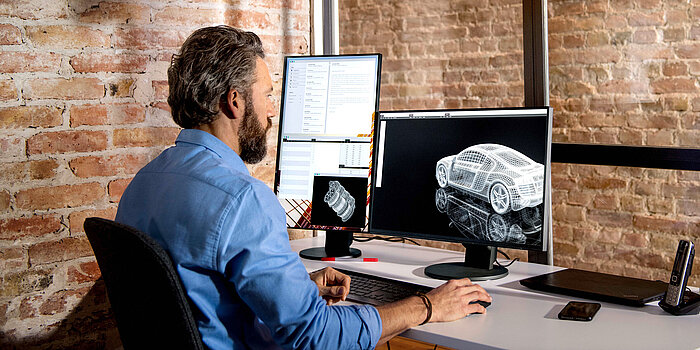A man with medium-length brown hair and a beard sits at a light-colored desk, which is white, in a room with exposed brick walls. He is positioned slightly to the left of center in the image, facing away from the camera and to the right. He is wearing a blue long-sleeve collared shirt with the right sleeve rolled up midway to his forearm, and a black bracelet on his right wrist. He is working on a computer, holding a mouse with his right hand, while his left hand rests near a black keyboard. 

In front of him are two monitors: the one directly in front is horizontally oriented and displays a white wireframe 3D rendering of an Audi A8. The second monitor, to the left, is vertically oriented and shows some white content with a diagram in a black square at the bottom right. There is a black closed laptop and a cordless phone on its docking station on the desk to the right of the horizontal monitor. Additionally, a black tray or plate is positioned between the cordless phone and the monitor. He is seated in a black chair, with its backrest visible behind him. To his left, there is a window looking out onto another brick wall.